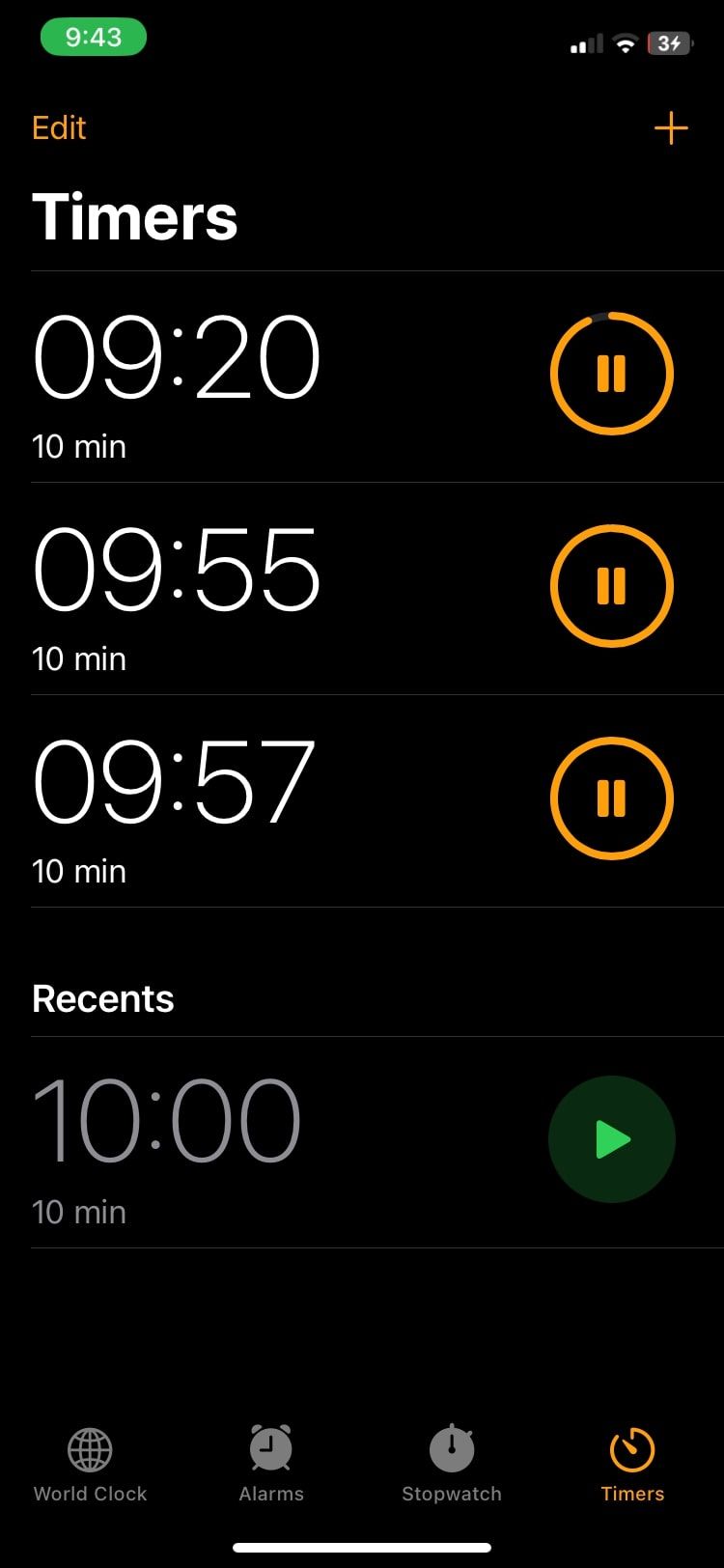The image captured from a smartphone features a vertically oriented interface with a solid black background revealing no texture or color gradient. In the upper left corner, there's a rounded green oval displaying the time '9:43' in white. Adjacent to it, on the right, indicators show the phone's signal strength, WiFi connectivity, and a low battery percentage of 3% with a charging icon.

Beneath the timestamp, the word 'EDIT' is highlighted in orange, flanked by a plus sign (+) on the right. Just below, in large, bold white letters, the word 'TIMERS' is displayed, separated by a dividing line. Below 'TIMERS', the display lists several active timers:

- The first timer reads '9:20' with a 10-minute duration. Opposite the time, there's an orange circular icon featuring a pause button.
- The second timer states '9:55', also with a 10-minute duration, alongside another orange pause button.
- The third timer shows '9:57' with the same 10-minute length, yet again aligned with a pause button icon.

Underneath the last timer, the section marked 'RECENTS' lists:

- '10:00' with a duration of 10 minutes, aligned with a green triangular play button.
  
At the bottom of the screen, navigational options 'Clock', 'Alarms', 'Stopwatch', and 'Timers' are visible, with 'Timers' illuminated in orange, indicating the selected mode.